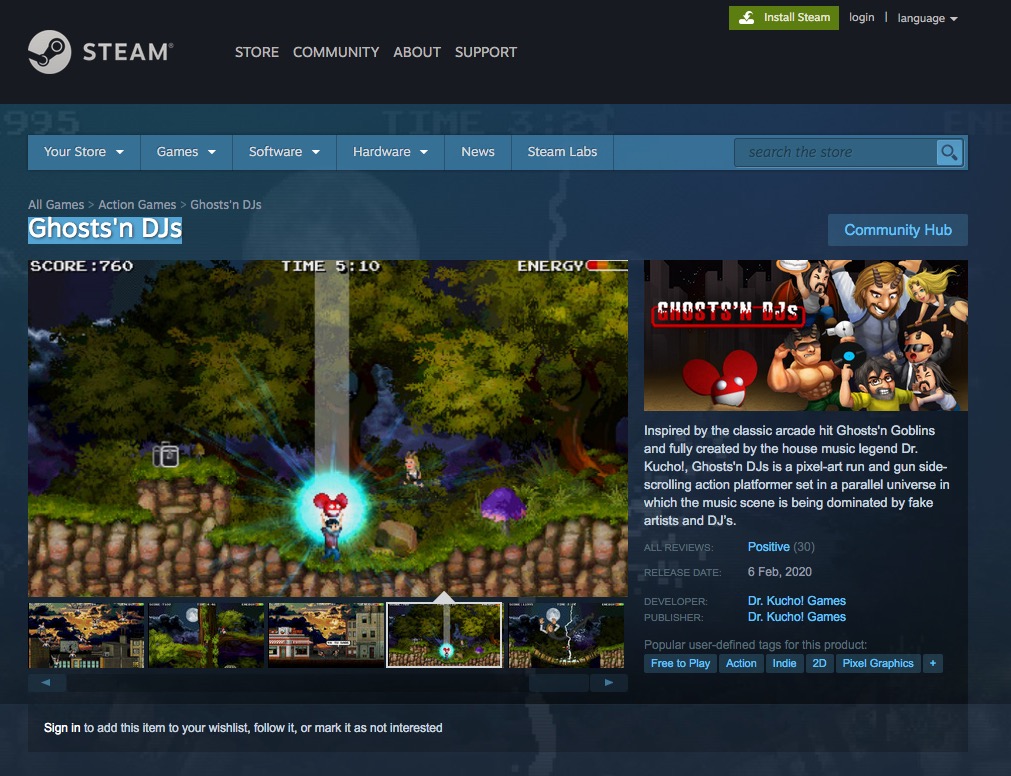This is a detailed caption for the image, cleaned up and formulated:

---

This is a screenshot from a website with a black background at the top. Prominently displayed is the Steam logo in white, accompanied by a circular icon featuring the recognizable Steam swirl. The header also includes options for "Store," "Community," "About," and "Support," along with a green "Install Steam" button. The user interface language option and login icon are also present.

Below this, a blue background ushers in the next section featuring tabs for "Your Store," "Games," "Software," "Hardware," "News," and "Steam Labs," as well as a search bar for the store.

Central to the screenshot is an image promoting the game "Ghosts, Indie, TJs." The image depicts a cartoon character situated in the middle of a forest, standing on the edge of a cliff. The character appears to have arrived via a beam of light emanating from above, encircled by a vibrant blue light. The game's interface displays a score of "760" at the top and a time of "5:10," with an energy bar located on the right side.

Adjacent to this, another image shows multiple characters, hinting at a diverse cast. The text indicates that the game is "inspired by the classic arcade Ghosts 'n Goblins" and "fully created by house music legend Dr. Kumu." The game, described as a "pixel art, side-scrolling action platformer," is set in a parallel universe where the music scene is dominated by fake artists and DJs.

Further information underlines the developer and publisher as Dr. Kumu Games, and the game's release date is listed as February 6th, 2020. Lastly, a sign-in prompt is visible in the bottom left-hand corner.